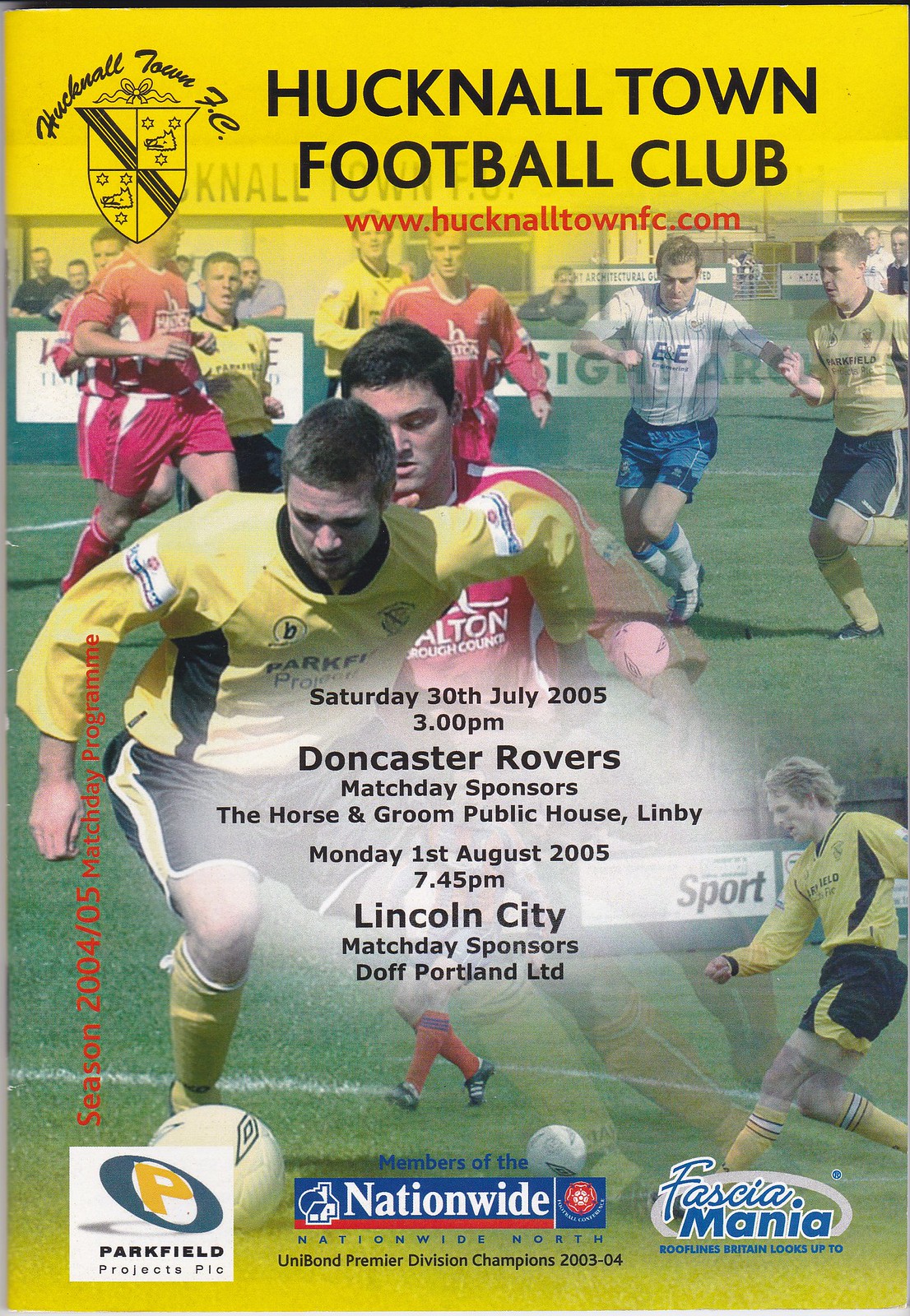The image appears to be the cover of a magazine or program advertising a series of football matches. Dominating the top section, a yellow banner hosts the name "Hucknall Town F.C." in black cursive and bold print, followed by "Football Club" and the website "www.hucknalltownfc.com" in small red font. To the left, a black shield with four diagonal sections displays boar head symbols and stars. Below the banner, the central image features a soccer pitch filled with players in various uniforms against a blurred background, suggesting a photoshopped composition. The diverse array of players includes individuals in blue, white, yellow, red, and black kits. In the foreground, two Caucasian players are vying for the ball—one dressed in yellow and black, the other in red and white. Event details are prominently displayed: "Saturday 30th July 2005, 3 p.m., Doncaster Rovers, Match Day Sponsors: The Horse and Groom Public House, Lindby," and "Monday 1st August 2005, 7.45 p.m., Lincoln City, Match Day Sponsors: Doff Portland LTD." At the bottom, sponsor logos appear: a blue circle with a yellow "P" for Parkfield, a blue background with white lettering for Nationwide, and a blue font outlined in white for Fastia Mania. The entire scene is set on a vibrant, green soccer field with additional spectators standing behind a distant wall.